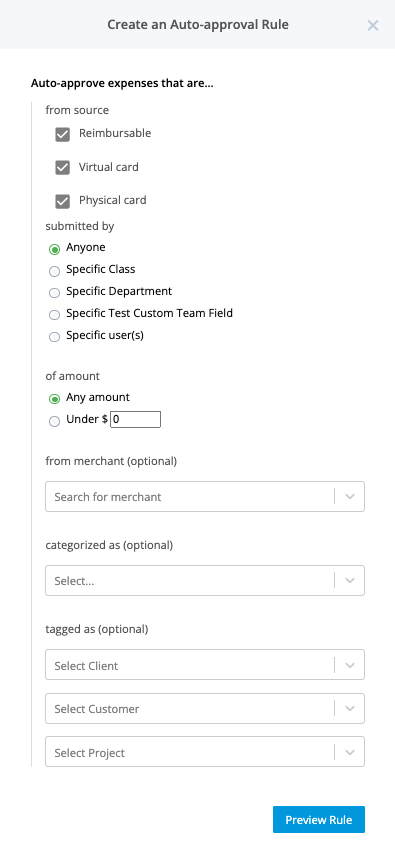The image is a screenshot of a webpage designed for setting up an expense auto-approval rule. At the top of the page, there is a semi-opaque gray bar with the title "Create an Auto-Approve Rule" and an 'X' on the right to close the window. Below this title, there is a section labeled "Auto-approve expenses that are from source" with three checkboxes: "reimbursable," "virtual card," and "physical card," all marked with gray check marks.

The next section is denoted by the label "submitted by" and features five multiple-choice options. Each option has a corresponding selection dot, and the option "anyone" is chosen, indicated by a green selection button. The five choices listed are: "anyone," "specific case," "specific department," "specific test," "custom team field," and "specific users."

Following this, there's a segment labeled "of amount," which also includes multiple-choice selections. The two options here are "any amount" and "under," with a fillable box for specifying an amount. The "any amount" option is currently selected.

Next are several optional dropdown boxes labeled: "from merchant," "categorized as," and "tagged as." The "tagged as" dropdown offers further options to select a client, customer, or project.

Finally, at the bottom-right corner of the screenshot, there is a blue box labeled "Preview Rule."